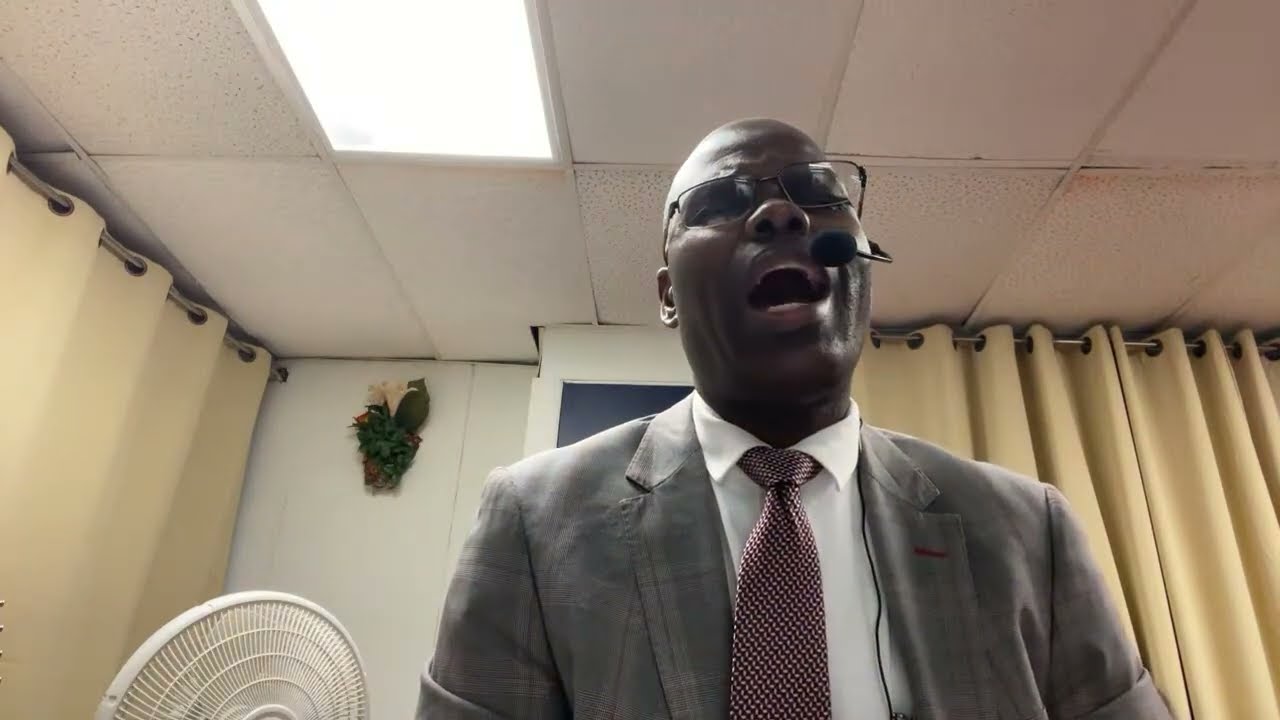In this detailed photo, an African-American man is captured from a low angle that showcases him from the chest up, placing him prominently near the center and occupying about one-third of the frame. The man is dressed in a light gray plaid suit, paired with a white dress shirt and a dark red tie adorned with small white specks. He wears glasses with metal frames and a hands-free microphone attached behind his left ear, featuring a black fuzzy ball windscreen.

The setting appears to be indoors, characterized by cream-colored, possibly gold or beige, curtains that drape from the floor to the ceiling, and white panel ceiling tiles above. Overhead, panel ceiling lights illuminate the scene. A white freestanding fan with its circular cage of blades is visible just behind him.

The man’s eyes are either shut or nearly shut, and his mouth is wide open, displaying an intense expression that suggests he might be speaking, singing, or preaching. The backdrop also includes a floral arrangement on what seems to be the far wall, consisting of small roses, a white tulip, and some vines, adding a decorative touch to the otherwise neutral setting.